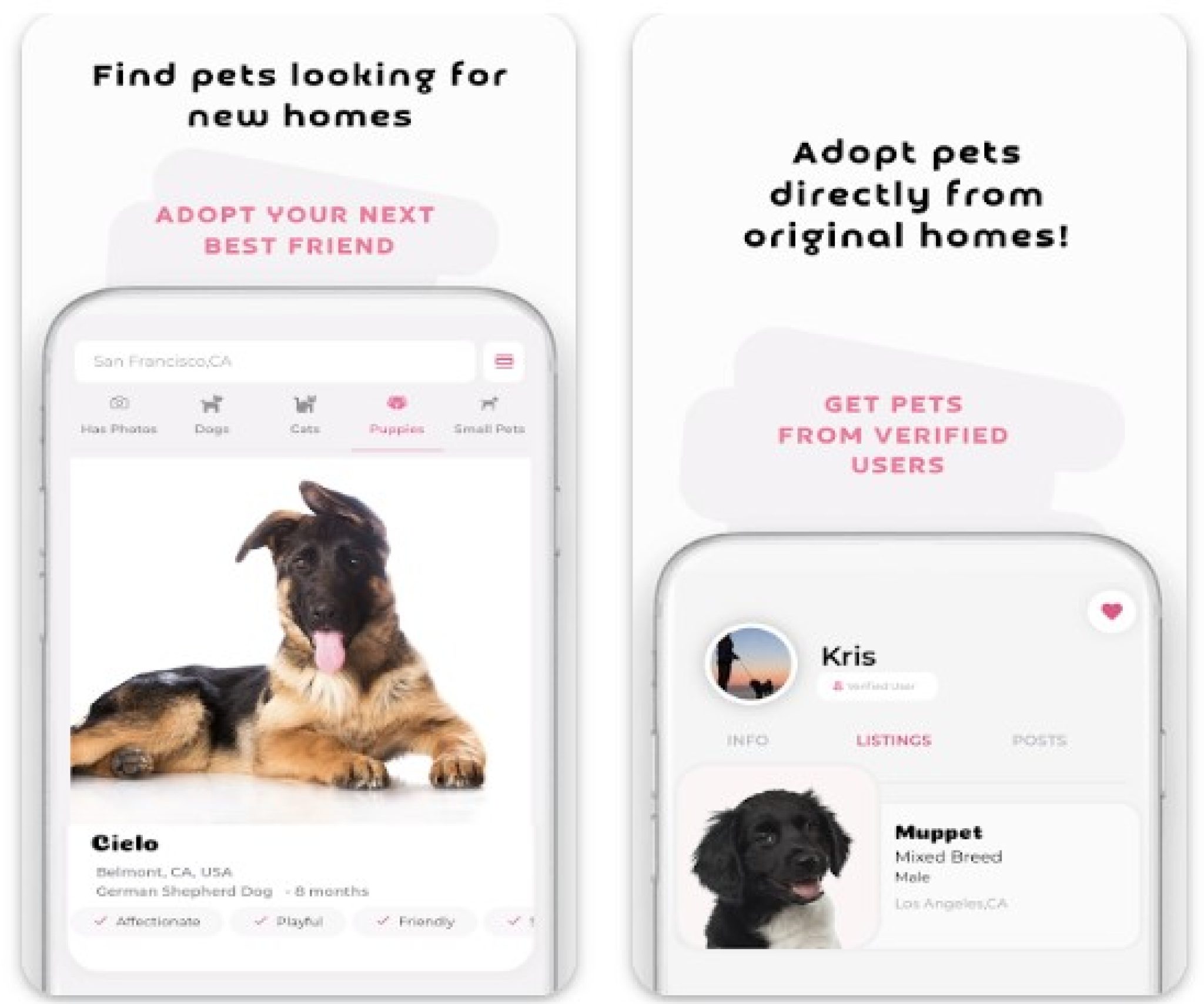The image depicts two advertisements side by side, promoting pet adoption through a mobile interface.

**Left Advertisement:**
- The header in bold black text reads, "Find pets looking for new homes," followed by a subheader in pink, "Adopt your next best friend."
- The interface displayed resembles a smartphone, with "San Francisco, CA" in a white box at the top.
- Multiple tabs are visible, labeled "Photos," "Dogs," "Cats," "Puppies," and "Small Pets."
- A prominent picture of a dog is featured. The dog has a black face and back with various shades of brown covering its body. It is sitting on its side with its tongue out.
- Underneath the image, black text reads "Cielo, Belmont, CA, USA." Additional details include "German Shepherd Dog, 8 months" and descriptors such as "Affectionate, playful, friendly."

**Right Advertisement:**
- The main message in bold black text states, "Adopt pets directly from original homes," with a secondary message, "Get pets from verified users."
- This section also features a phone interface.
- At the top appears the name "Chris" and a small silhouette of a person walking a dog, accompanied by a heart icon in the top right corner.
- Below, tabs are labeled "Info," "Listings," and "Posts."
- A picture of another dog is showcased with a black face and a white chest, its mouth open as if panting.
- The text under the image reads, "Muppet, Mixed Breed, Male, Los Angeles, CA."

This detailed image caption delivers a comprehensive understanding of the advertisements, emphasizing the variety of adoptable pets and the primary features of the mobile interface.